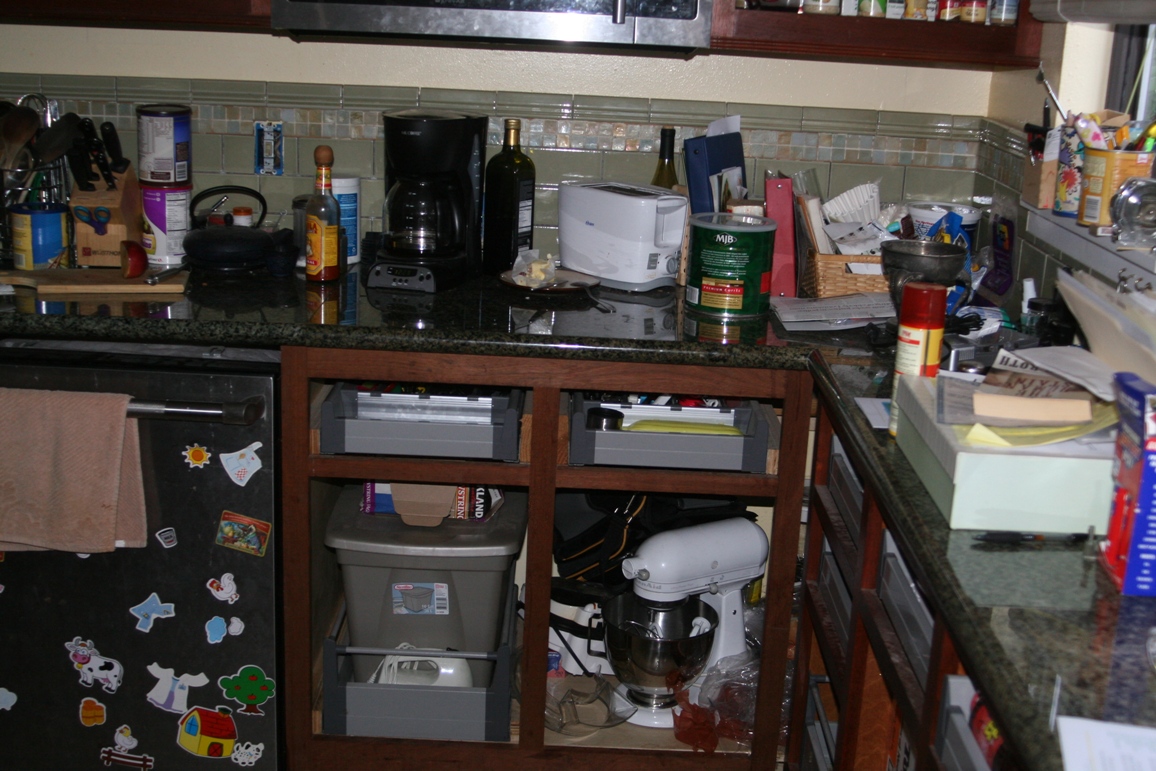This image captures a bustling kitchen space featuring a dark mahogany L-shaped countertop adorned with a variety of household items. The countertop, made of dark granite, sets a rich and elegant tone for the kitchen, but the scene is lively and somewhat cluttered.

Starting from the left, a dishwasher decorated with whimsical children's stickers such as cows, houses, trees, and suns immediately catches the eye. A peach-colored towel is neatly draped over the bar of the dishwasher door. Above the dishwasher, a knife block holding a set of black-handled knives is surrounded by an assortment of cans.

Moving right along the countertop, a bottle of Cholula hot sauce sits next to a traditional glass coffee maker. Nearby, a glass oil bottle, a white toaster, and a large, unidentifiable coffee can add to the diverse assembly of items.

The backsplash behind the countertop features olive-green tiled walls that complement the darker cabinetry. Interestingly, the cabinets below lack doors, leaving the contents visible. The drawers too are exposed, revealing a more rustic and unpolished look. 

On the far right, clutter dominates the scene with a bread binder, possibly a recipe book, and a wicker basket filled with coffee filters. There are some additional books stacked closer to the right-hand side, near the small windowsill which is also laden with cans.

Overall, this kitchen scene, though organized in some parts, reflects a busy and lived-in space full of character and daily life.